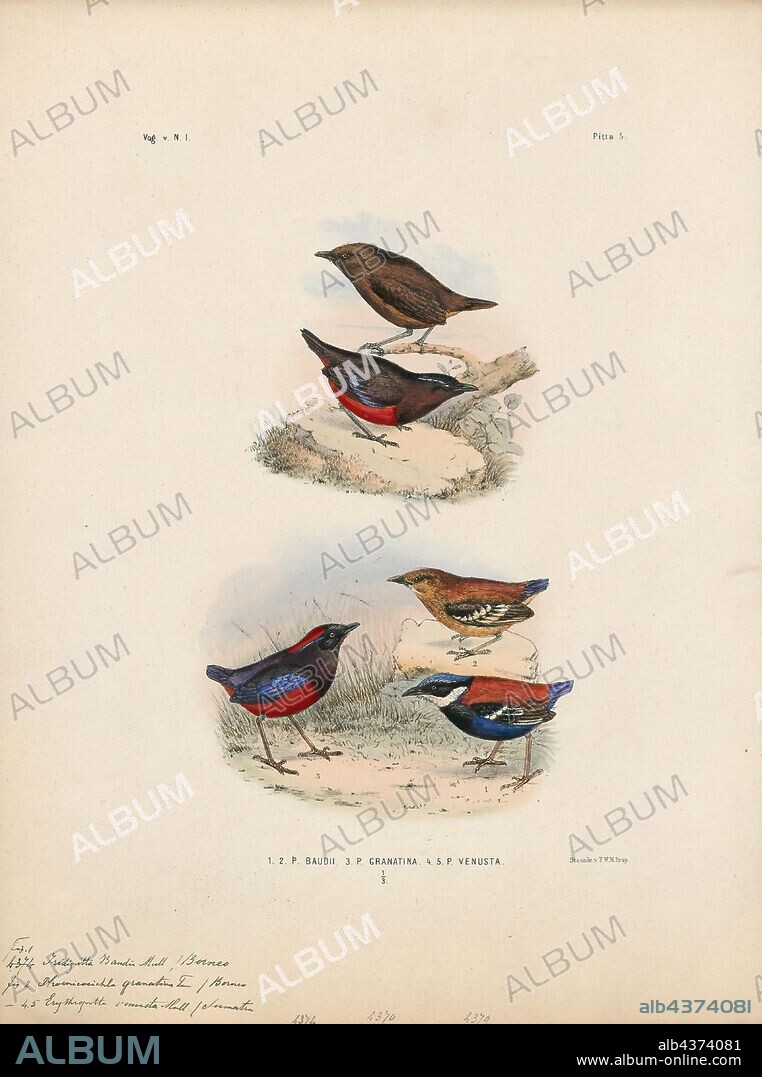The image features multiple detailed illustrations of various finches, showcasing a blend of colors including brown, red, blue, and black. The illustrations are arranged into two distinct groups. In the top section, one small bird is entirely brown and perched on a branch, while the other has a darker brown head and bright crimson red belly, and stands on the ground. Below them, the grouping includes a bird with a red belly, blue wings, and red head, alongside another with a red back, blue belly, blue head, blue tail, and a white jaw and neck. The final bird in this section is perched on a rock, characterized by its brown body, blue tail, and black beak. The cream-colored background of the image has multiple watermarks with the word "album" and additional scattered handwriting. The bottom of the image features a link to a website, www.albumonline.com, suggesting the images may be associated with the Audubon Society, possibly indicating bird species observable in certain regions. The use of the word album repeatedly hints at the collection's formal presentation or perhaps a form of copyright marking.